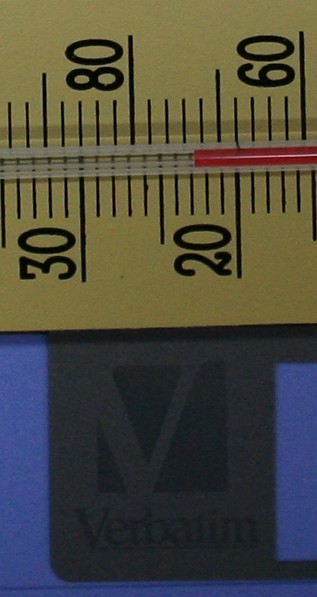A peculiar image featuring a sideways thermometer juxtaposed with a 'Verbatim' logo, both set against a background that resembles a blue binder or a floppy disk. The thermometer registers approximately 73°F (23°C), with both Fahrenheit and Celsius scales visible. The 'Verbatim' logo, typically associated with office products, adds to the odd pairing. The overall composition is somewhat ambiguous, blending elements that evoke nostalgia and practicality.